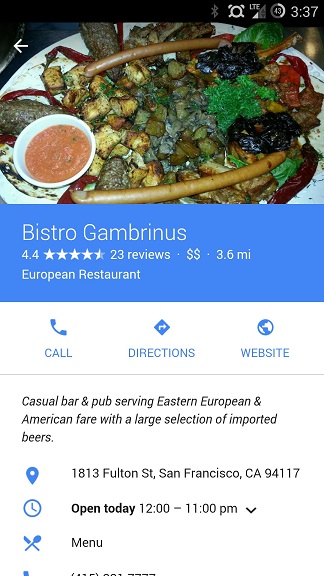On a plain white background, the time is displayed as 3:37 alongside a Bluetooth symbol. The central focus of the image is a plate of food, featuring what appears to be potatoes and possibly lamb meat. Also included in the image is detailed information about a restaurant named Bistro Gambrinus, which boasts a rating of 4.4 stars from 23 reviews. The restaurant is located 3.6 miles away and is categorized under European cuisine. Additional text indicates that besides being a European restaurant, it is a casual bar and pub offering Eastern European and American fare, and known for its extensive selection of imported beers. The establishment's address is listed as 1813 Fulton Street, San Francisco, CA 94117. The operating hours are noted as open today from 12 PM to 11 PM. An arrow suggests there may be more options such as viewing the menu, although the phone number present is cut off midway.